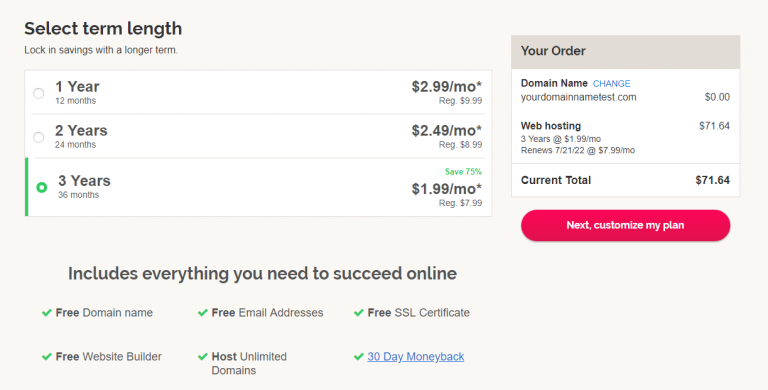The image displays a webpage where users can purchase domain names and web hosting services. The pricing options are structured based on the duration of the subscription. The service offers three terms: one year at $2.99 per month (regularly $9.99), two years at $2.49 per month (regularly $8.99), and three years at $1.99 per month (regularly $7.99). The three-year term, which saves 75%, is selected as indicated by a green button.

The order summary outlines the details, including the domain name "yourdomainnametest.com," with an option to change it via a blue hyperlink button. The domain name costs $0. For web hosting, the selected term is three years at $1.99 per month, which will renew on July 21, 2022, at $7.99 per month, totaling $71.64 for the duration. The current total payment due is $71.64. A red button labeled "Next: Customize My Plan" invites users to proceed with customizing their plan.